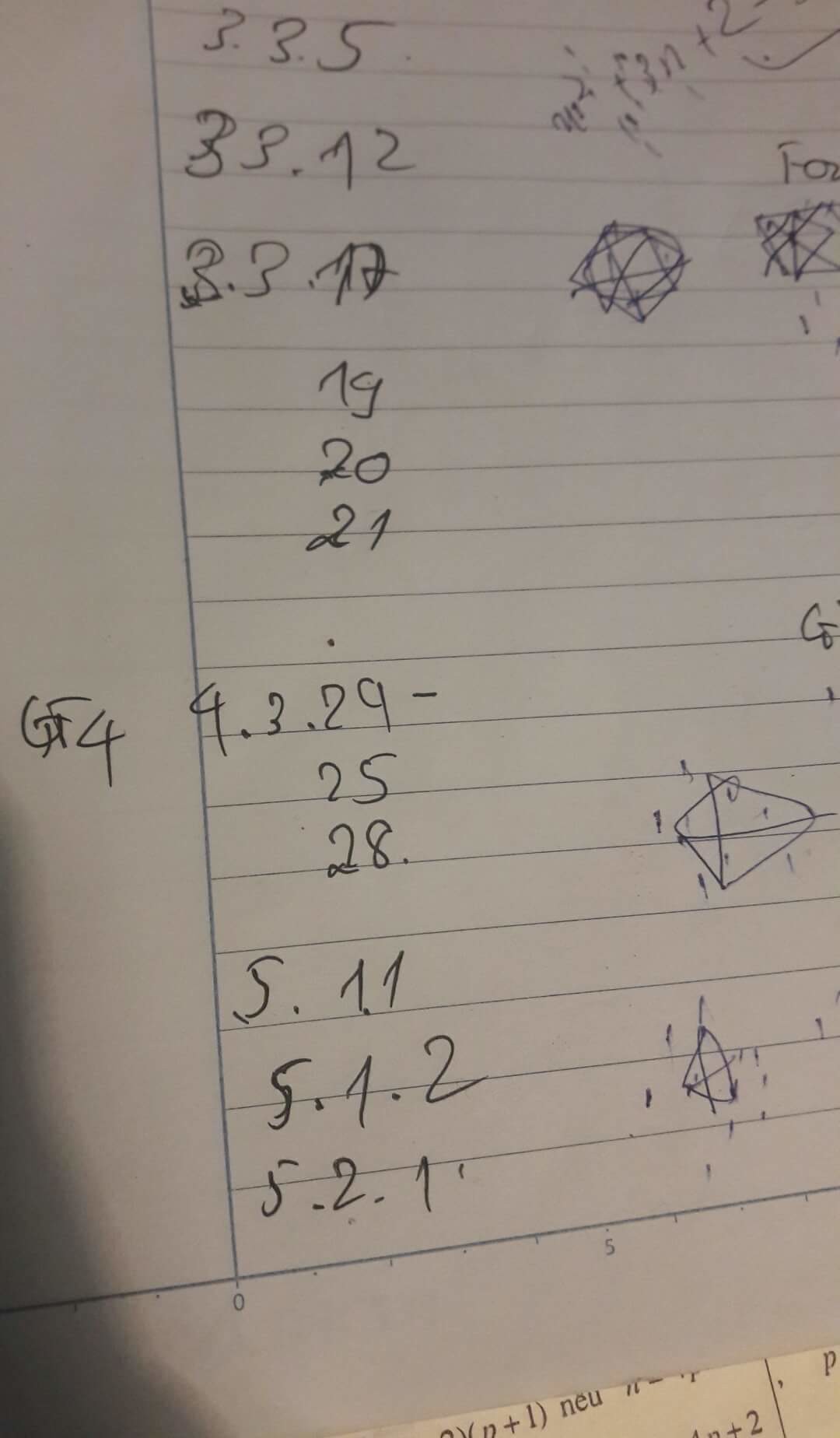The image depicts a sheet of paper with wide-ruled lines, half of which is lined while the column on the left side is unlined. No written paragraphs are present, but the page is filled with mathematical notations and symbols, indicating someone might be working on math problems. In the unlined section on the left, the notation "GF4" is conspicuously written and stands out on its own. Alongside this, the lined section contains numerical sequences “33.5,” “33.72,” “33.72,” and continues similarly down the page, each set separated by a skipped line. Further down, the numbers “90” and possibly “43.29” appear in the same staggered format. Toward the bottom, there are consecutive entries like “S.11,” “5.4.2” (or possibly another variation if a numeral is misread), and “5.2.1.” At the very bottom edge, some printed text is visible, which appears to be made from a textbook. Additionally, various geometric designs are scattered across the page, adding to the sense of mathematical exploration and sketching.